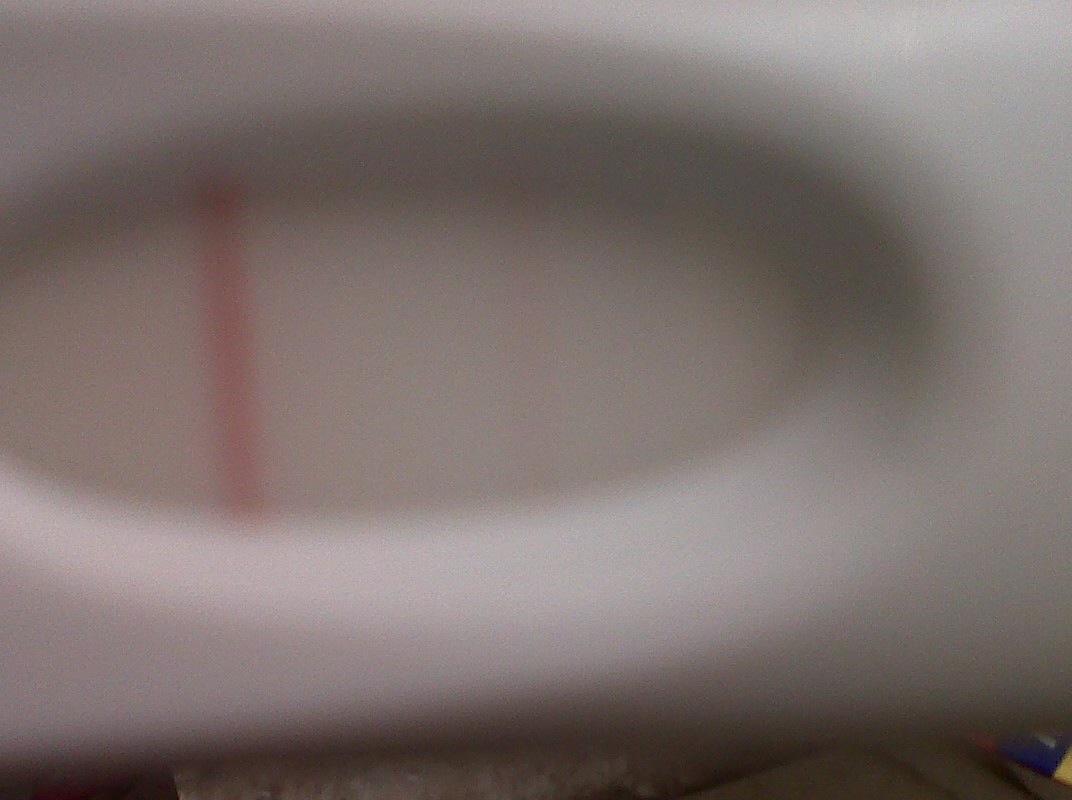The image depicts a close-up, highly blurred view of a test kit, which could be either a COVID test or a pregnancy test. The test device is white, featuring an oval window with two vertical lines inside it. One line is distinctly colored in pink or red, while the other line is faint and almost transparent, yet still visible. Surrounding the test kit are various background elements, including a brown object, a white object with hints of pink, and another item displaying blue, red, and yellow hues. The ambiguity of the setup is emphasized by the lack of a readable chart or labels, leaving the test's purpose and result indeterminate. The overall appearance and context leave viewers uncertain about the specific nature and outcome of the test.